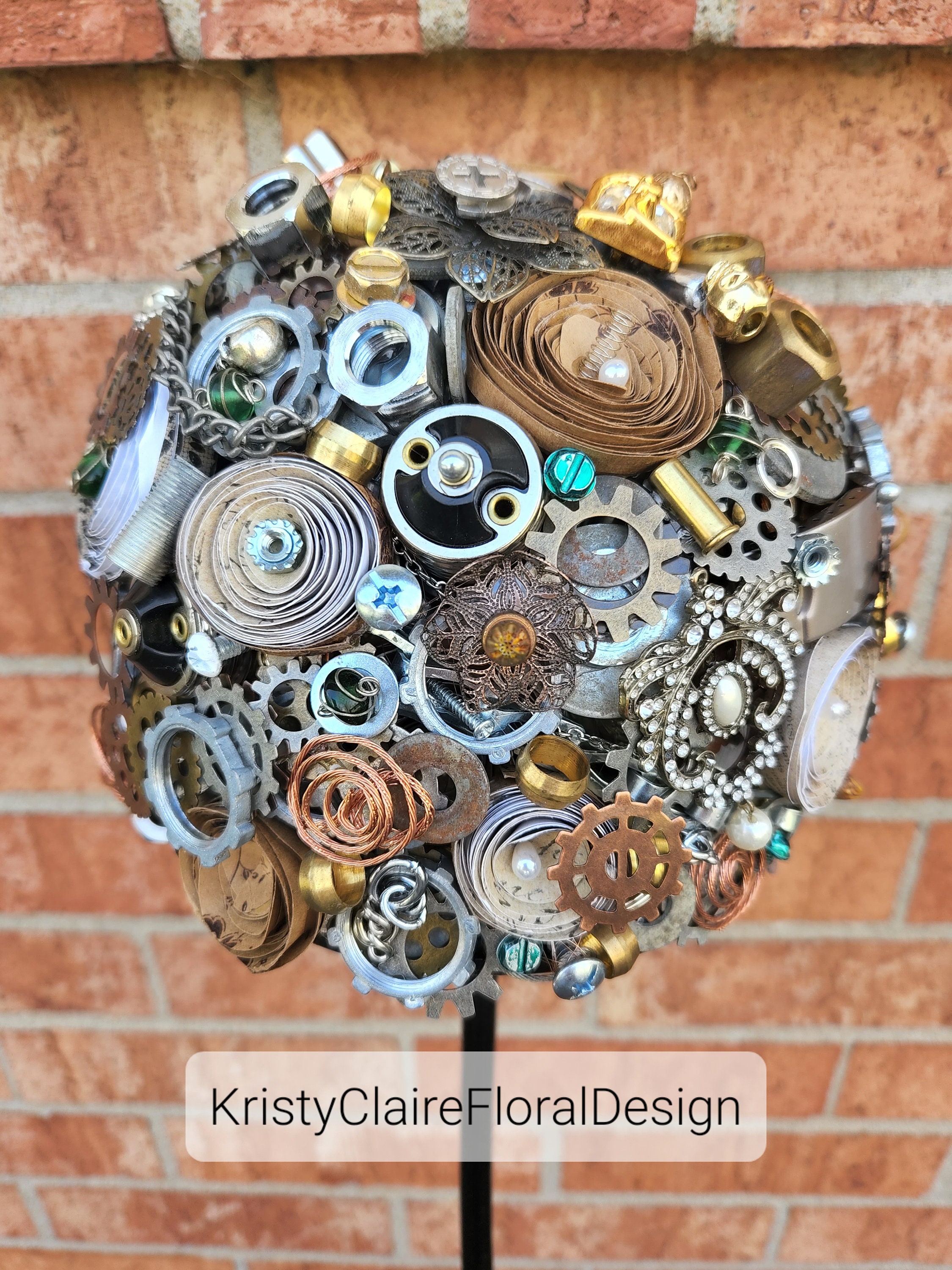This photograph showcases an impressive and detailed piece of modern art, meticulously crafted from various metallic objects, including gears, nuts, bolts, wrenches, chains, and even small pieces of jewelry like brooches. The art piece is designed to resemble a large, intricate floral ball where elements of metallic flowers are notable, complete with circular petals and colorful, central components. The metals exhibit a palette of colors, including shades of copper, silver, gold, blue steel, and some green, adding to the visual complexity and richness of the artwork. This floral sculpture is mounted on a black pole and set against a neutral red brick wall backdrop, which enhances the focus on its fine details and craftsmanship. At the bottom of the image, digitally added text displays the username "Christy Clare Floral Design" in black letters within a semi-transparent white-bordered rectangle, suggesting this photo likely serves as a promotional piece for social media or a website.